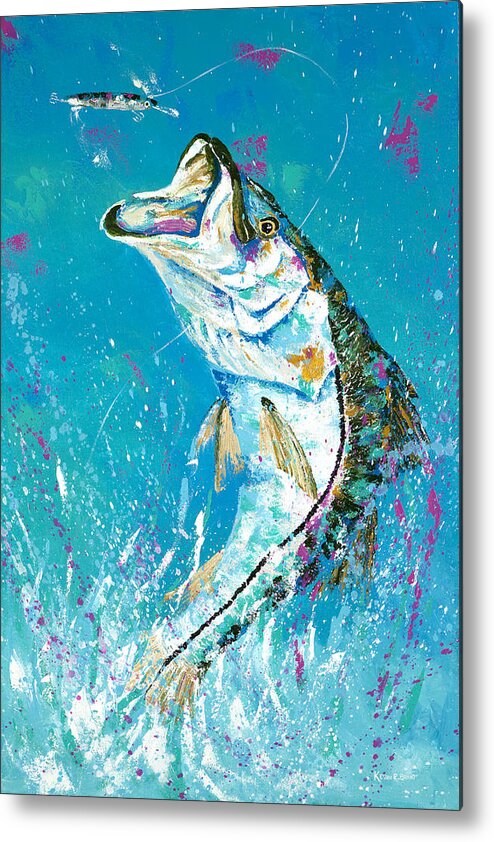This whimsical image, resembling a CGI creation or a vibrant painting, captures a dynamic scene of a largemouth bass leaping out of the aqua blue water, mouth wide open to catch what appears to be a bait at the end of a barely visible fishing line. The fish, tilted slightly to the left, boasts a white belly adorned with blue and yellow markings, and a colorful interior of pink and yellow hues. Its back and fins have hints of green, and a striking yellow eye completes its spirited appearance. The backdrop features splashes of purple and green with white streaks that indicate the motion of the fish's powerful jump, adding to the fantastical quality of this captivating aquatic moment.